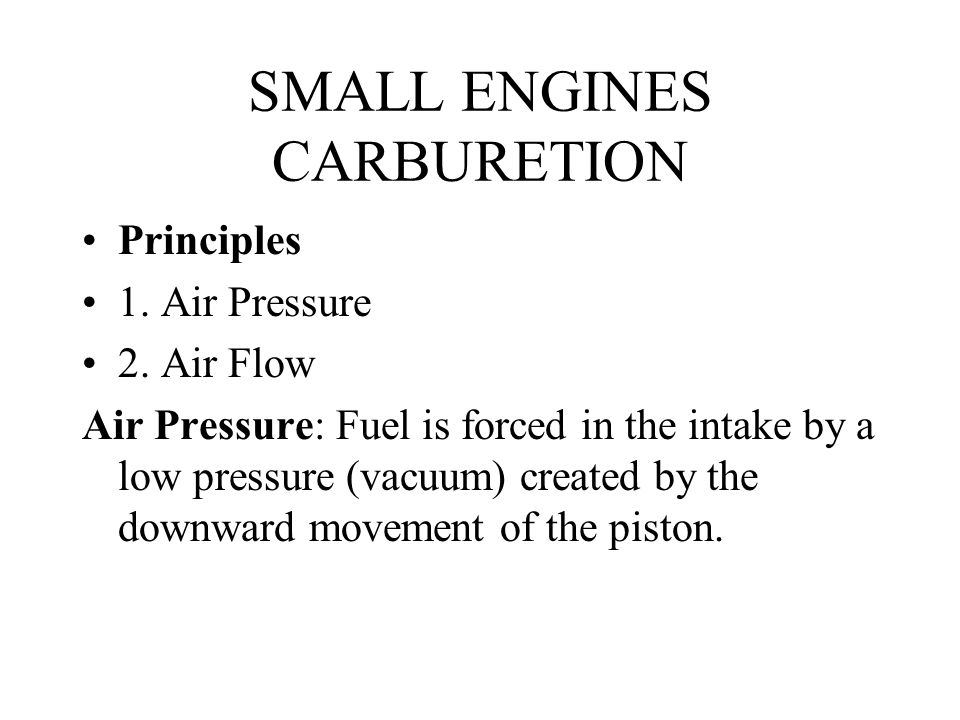The graphic features a simple, text-only design on a white background with black text. At the top center, the title reads "Small Engines" on the first line and "Carburetion" on the second line. Below this, there are three left-aligned bullet points. The first bullet point, in bold, is labeled "Principles." The second and third bullet points number "1. Air Pressure" and "2. Airflow," respectively. Further down, in bold, is the phrase "Air Pressure:" followed by a definition that reads, "Fuel is forced into the intake by a low-pressure (vacuum) created by the downward movement of the piston." This concise, informational card appears as though it could be a summary slide from a Google presentation or a page from a textbook or instruction manual, providing a clear and focused overview of key concepts in small engine carburetion.